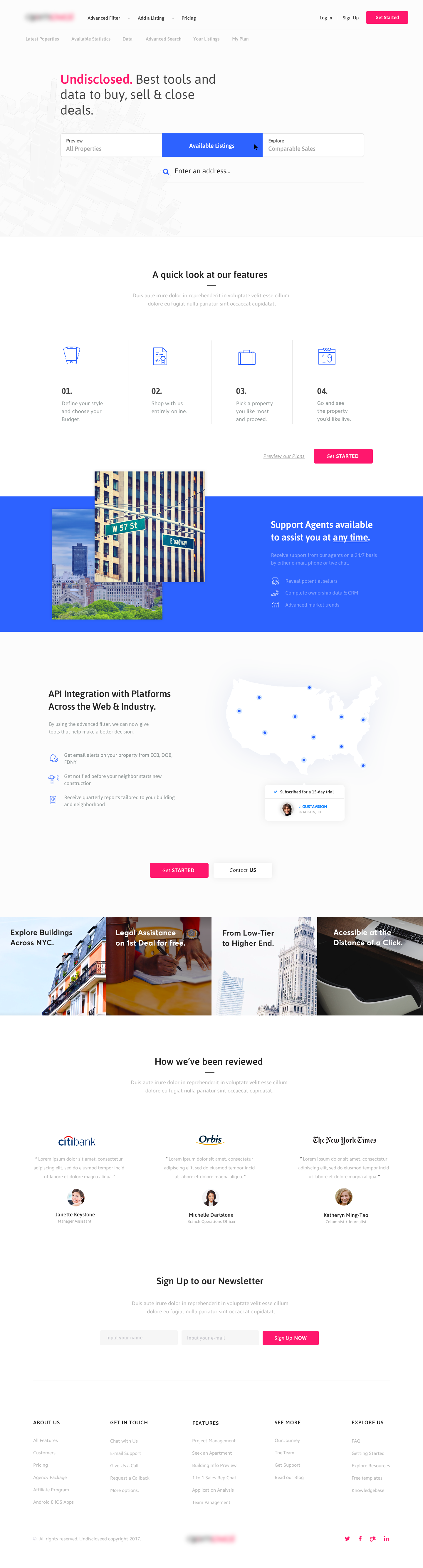This image showcases a webpage with a clean, white background. In the upper left corner, there is a black and pink logo and the name of the website, though they are blurred out. At the top of the page, navigation tabs are displayed on the left and right sides, with a prominent pink button in the far upper right corner.

Beneath the navigation bar, there is a section titled "Undisclosed Best Tools and Data to Buy, Sell, and Close Deals." This section features a box for inputting information, accompanied by a blue button.

Further down, a heading reads "A Quick Look at Our Features," followed by four blue logos or icons, each with explanatory text below. 

A blue box announces, "Support Agents Available to Assist You at Any Time."

The page also includes multiple images and a map. There is a section highlighting reviews with logos from Citibank and a company that appears to be named Osiris.

At the very bottom, there is an option to sign up for their newsletter.